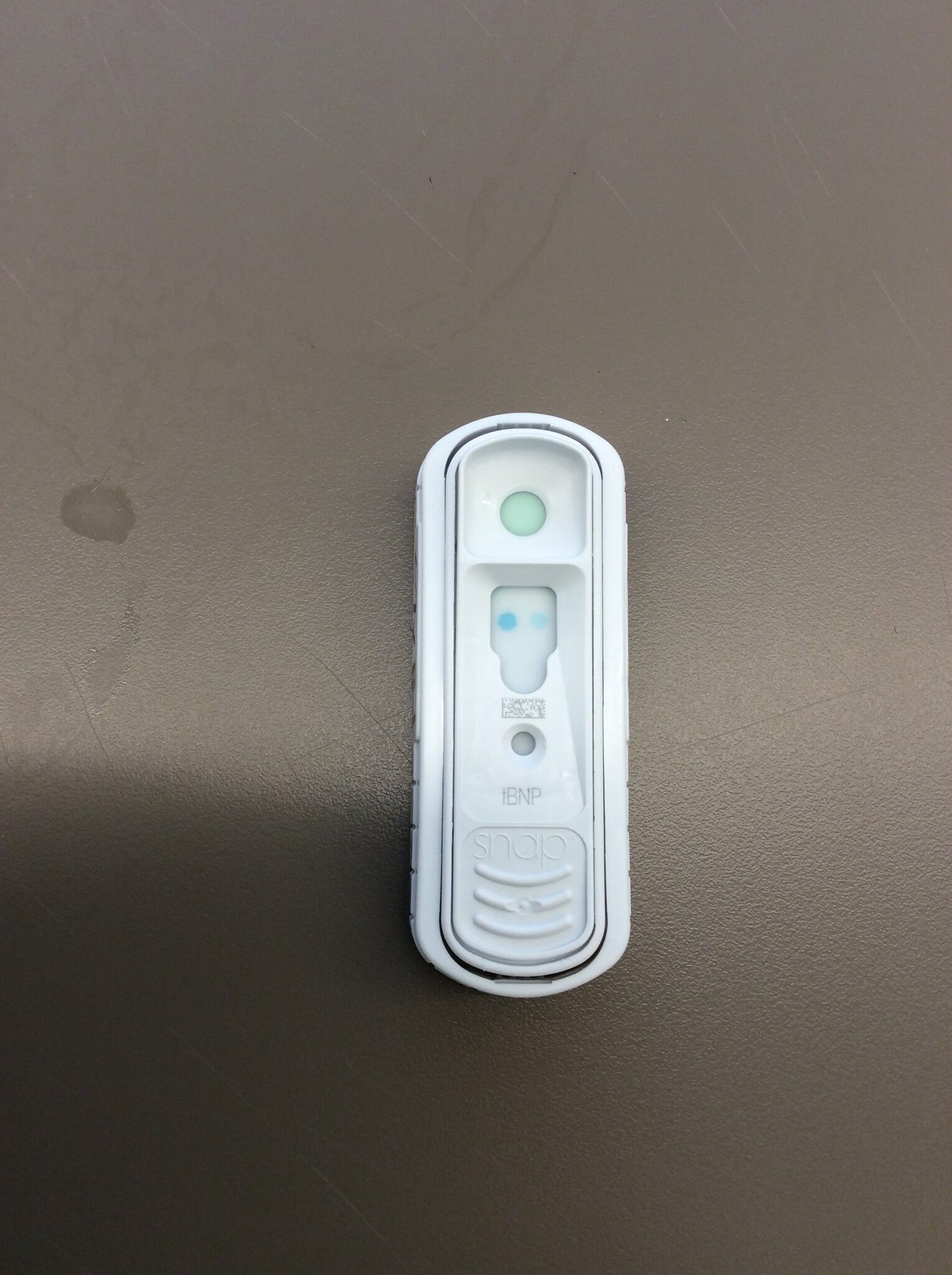This portrait-oriented photograph captures a small, white, plastic device resting on a medium gray, slightly scratched surface, likely a countertop. The device is centrally positioned within the frame and has a rounded top and bottom, forming a rectangular shape. 

In the very center of the object, there is a small hole. Positioned above this hole is a distinctive, square-shaped indentation housing two blue dots side by side, with the left dot being a darker shade of blue. Above this formation, there is another square indentation containing a tiny round shape inside. 

Beneath the central hole, the letters "IBP" are prominently displayed. Further down, the word "snap" is embossed in the same white plastic material, accompanied by three rounded lines below it. This object appears to be some sort of diagnostic test device, potentially designed to hold a liquid sample for analysis.